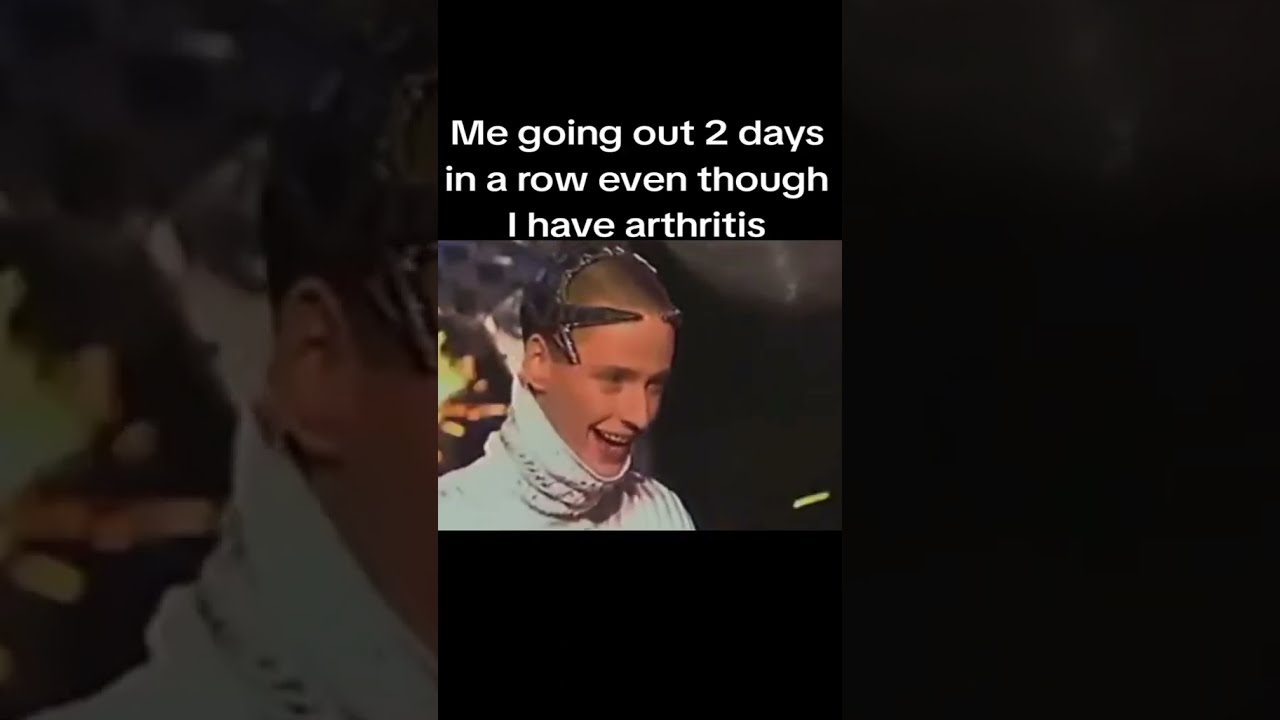In the center of a dark, black background, there is a small, somewhat blurred image featuring what appears to be flames or a burning building. In the foreground, prominently displayed, is a close-up photo of a smiling white Caucasian male with a shaved head, the top of which appears dark and shadowed. He is donning a white turtleneck that wraps snugly up to his chin, concealing his neck. Adorning his head is a peculiar contraption resembling a starfish, with points extending over his forehead on each side, giving the impression of a metal crown or headset clamped around his head. Despite the potentially painful situation, his expression conveys amusement, evidenced by the smile in his eyes. Overlaying this image, in white print, is the humorous caption: "Me going out two days in a row even though I have arthritis."